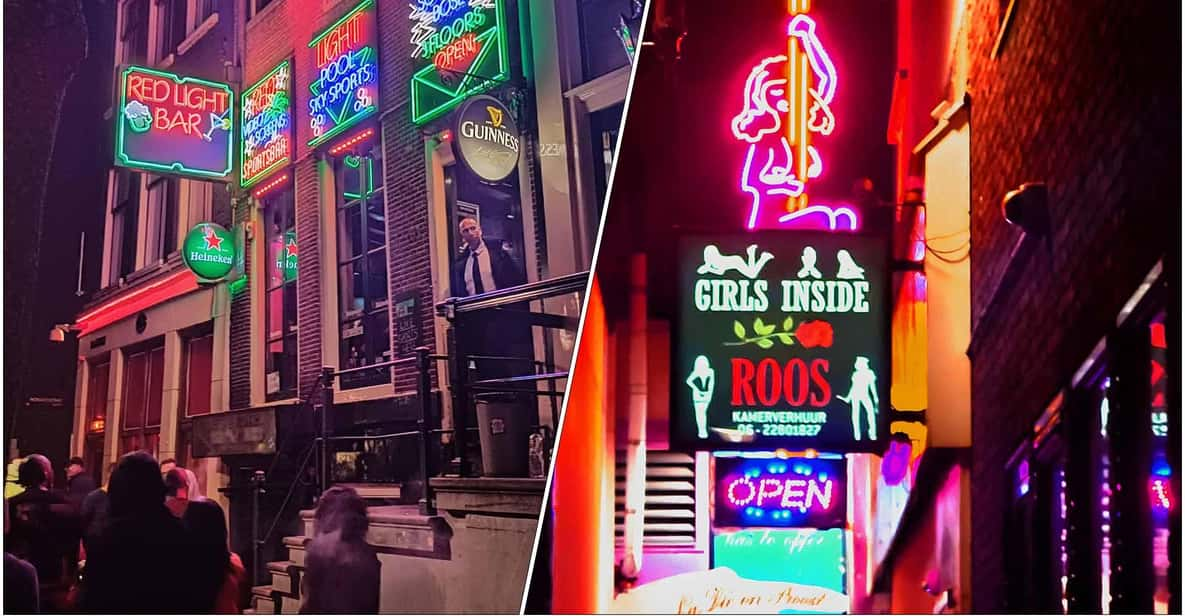This night-time outdoor composite photograph captures the lively essence of a city's red light district, split into two distinct yet related scenes. On the left side, a bustling brick building houses the Red Light Bar, prominently featured with red neon signage depicting a beer glass and a cocktail martini glass beneath it. Complementing this vibrant display are additional neon signs for Heineken and Guinness beers, along with advertisements for pool and Sky Sports, marked by a "Bar Sound by Bose" sign. Amidst these glowing lights, people can be seen milling around, with a notable figure standing in the doorway clad in a dark jacket, white shirt, and black tie. 

The right side of the image draws attention to a marquee for an adult entertainment venue. The neon sign reads "Girls Inside R.O.O.S," accompanied by a striking depiction of a partially clothed woman on a neon pole. Below this, another neon sign simply states "Open." This side of the split image, which is delineated by a diagonal white line, offers a view looking upwards toward the sky, emphasizing the brick buildings and the night-time setting free of any additional people.